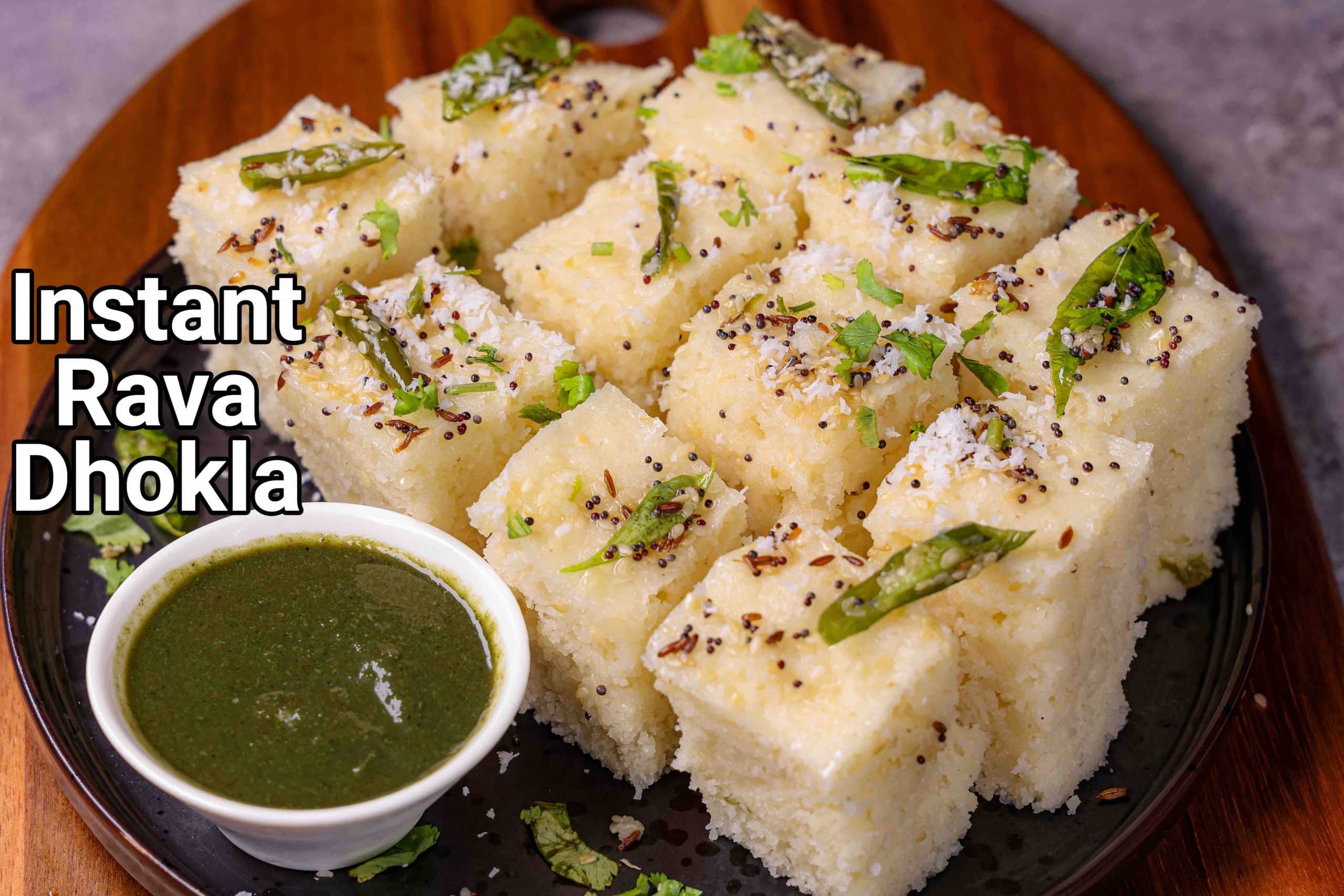This image showcases an authentic Indian dish called Instant Rava Dhokla, presented in a highly detailed and visually appealing manner. The Rava Dhokla, a light, spongy delicacy, is cut into 11 tall, beige cubes, arranged neatly on a sleek black ceramic plate. These cubes are garnished with brown spices, herbs, and small green leaves, resembling arugula or lettuce, adding both flavor and a touch of elegance to the presentation. Accompanying the dish is a small white cup filled with a thick, deep sage-colored dipping sauce, likely intended to complement the flavors of the Dhokla. The black plate is placed on a round wooden serving tray, which is set on a purplish-dark colored table or countertop. The words "Instant Rava Dhokla" are prominently displayed on the left side of the image in bold, white block letters with a black outline, suggesting the dish might be featured for a recipe or a tutorial. This detailed presentation captures the essence and intricate details of this delectable Indian treat.